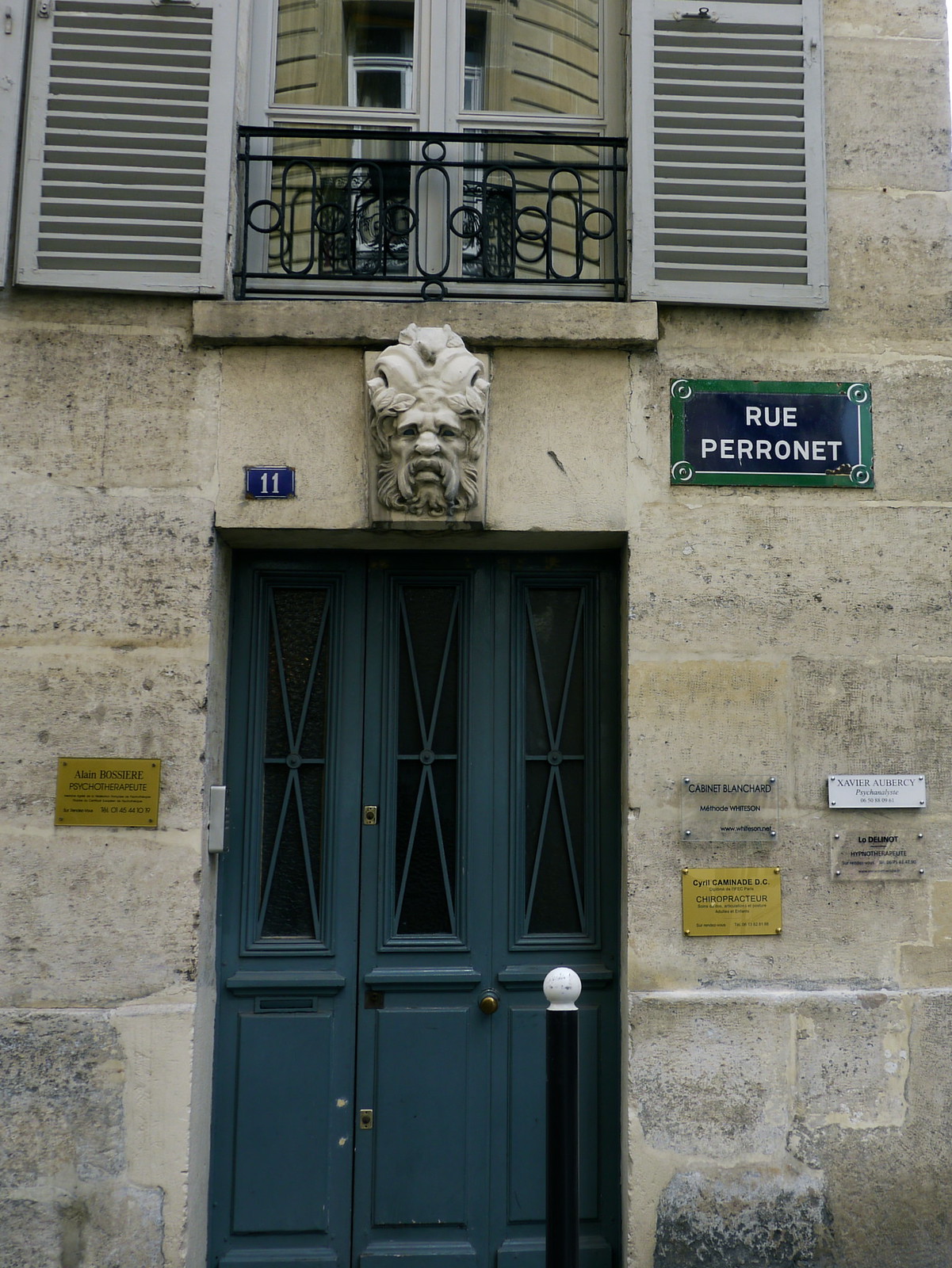This image depicts the exterior of a building constructed with large white bricks featuring gray and black marbling. Centered at the base of the image is a distinctive green door, adorned with three windows, each marked with green X-shaped designs. Above the door, a sculpted face of a man, bearing a lion-like appearance with a mane and warrior-like features, is affixed to the building. Flanking the door on either side are various gold and bronze plaques, detailing different professional practices within the building: “Alan Rosary Psychotherapist” to the left, “Cyril Skamene DC Chiropractor” to the right, along with “Cabinet Blanchard” and a reference to a hypnotherapist further right, and a silver plaque reading “Xavier Obercy Psychoanalyst” adding to the list. A blue number 11 sits above the door, alongside a blue and green sign with white text that reads "Rue Perronet," possibly indicating the street name. Higher up, the building features white shutters, a black metal railing, and windows that might suggest apartment spaces, adding to the complex facade of this multi-use structure.